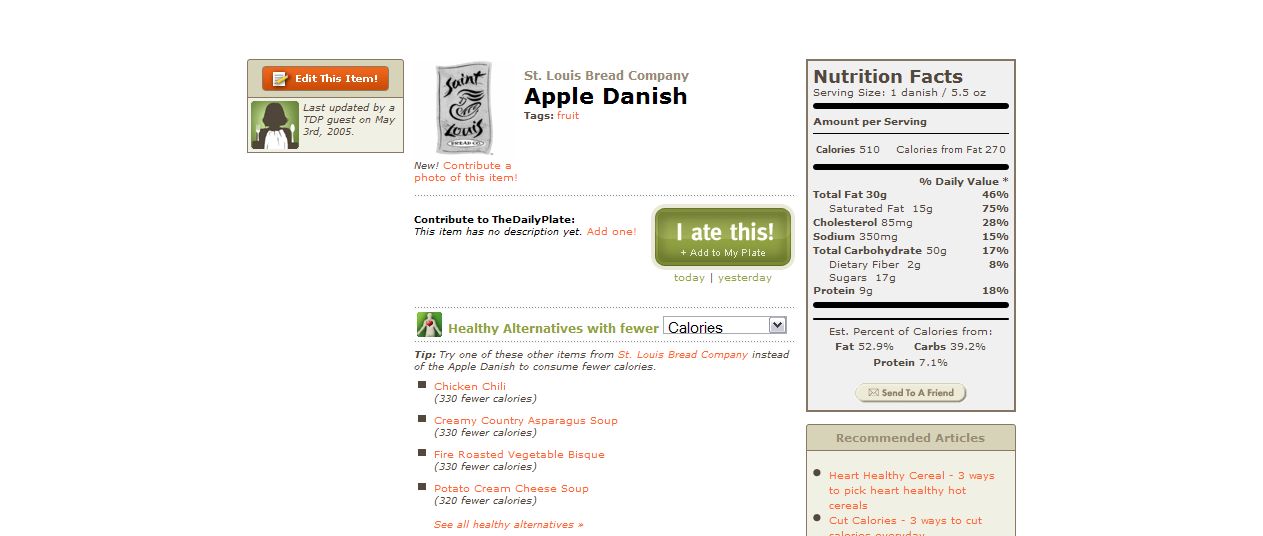This image is a detailed screenshot from a calorie tracking app or website, showcasing the item "St. Louis Bread Company, Apple Danish." The central portion of the image displays pertinent information: the product name, tagged as "Fruit," and indicates that it was last updated by a TDP guest on May 3, 2005. On the left side, there is a button labeled "Edit this item" within an orange rectangle, and below this is a teal rectangle with the update information. Adjacent to this, there's a small gray icon representing the St. Louis Bread Company, as well as a call to action to contribute a photo of the item or to contribute to "The Daily Plate," a feature presumably meant for adding or editing item descriptions.

The right section of the screenshot presents a detailed Nutrition Facts label with comprehensive dietary information. It lists the serving size as 1 Danish (5.5 ounces) with caloric content and macronutrients: 510 calories, 270 from fat, 30 grams of total fat (including 15 grams of saturated fat), 85 milligrams of cholesterol, 350 milligrams of sodium, 50 grams of total carbohydrates (including 2 grams of dietary fiber and 17 grams of sugars), and 9 grams of protein.

Additionally, there are features that include options like "I ate this, add to my plate," suggestions for healthy alternatives, and related articles on other items such as Chicken Chili, Creamy Country Asparagus Soup, Fire Roasted Vegetable Bisque, and Potato Cream Cheese Soup. The overall layout and details suggest a platform designed to give users a comprehensive overview and options to interact with and edit their dietary entries.